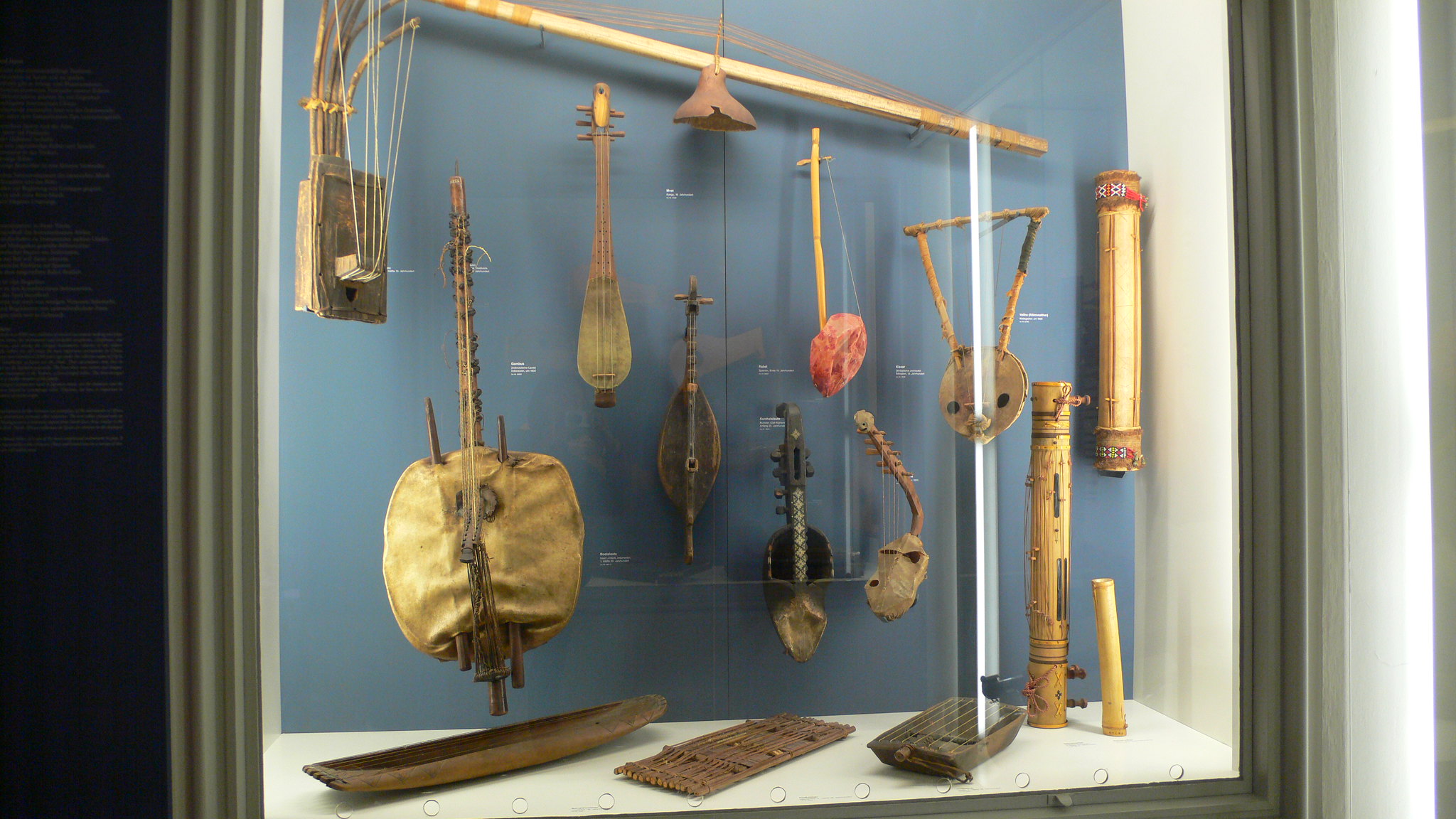This photograph captures a museum exhibit showcasing ancient musical instruments behind a glass case with a greenish-gray wooden frame. The back wall of the display is a medium blue-gray shade, providing a contrasting backdrop to the white side walls and base of the case. Suspended from a brownish-gold rod near the ceiling, several strings hold a variety of weathered, primitive instruments. Among these are a broken bell, a rectangular stringed instrument, and a mandolin-shaped piece, all hinting at their historical and musical significance. The collection includes a mix of shapes and sizes, with a notable instrument resembling a violin, and an assortment of rain sticks and items intended for percussive use scattered at the base. The craftsmanship and age of these wooden instruments, some featuring attached sacks or bellows, imbue the display with an aura of ancient musical heritage.